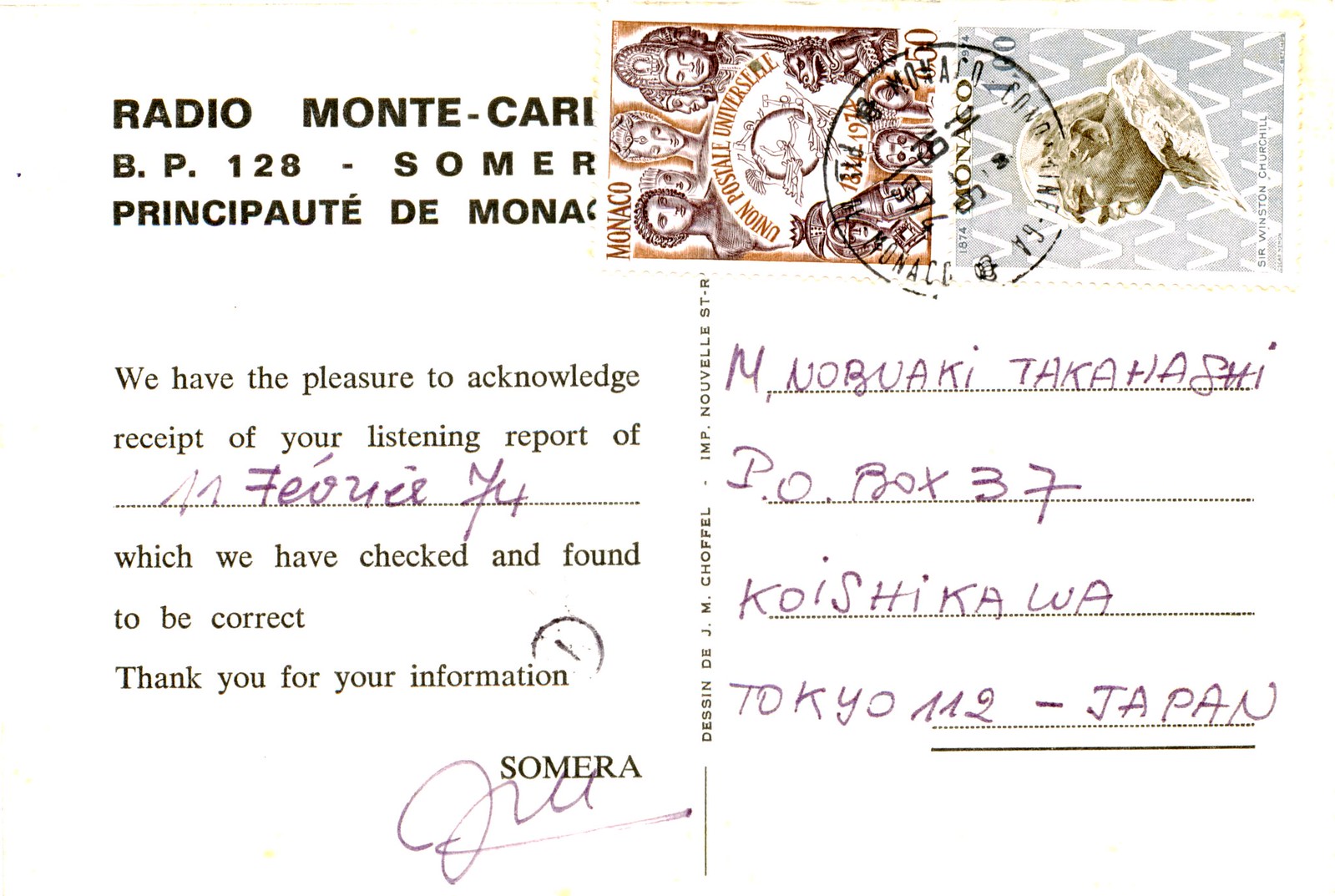The image appears to be a scan of a postcard sent from the Principality of Monaco, specifically Radio Monte Carlo, to Nobuaki Takahashi at P.O. Box 37, Koishikawa, Tokyo, Japan. The left side of the postcard, written in black text, acknowledges receipt of Mr. Takahashi's listening report, noting that it has been checked and found to be correct. The text reads, "We have the pleasure to acknowledge receipt of your listening report of [name filled in], which we have checked and found to be correct. Thank you for your information. Somera." The right side features the handwritten address to Mr. Takahashi, along with two postage stamps and a postmark. This postcard serves as a confirmation from Radio Monte Carlo to Mr. Takahashi in Japan, indicating the accuracy of his report.